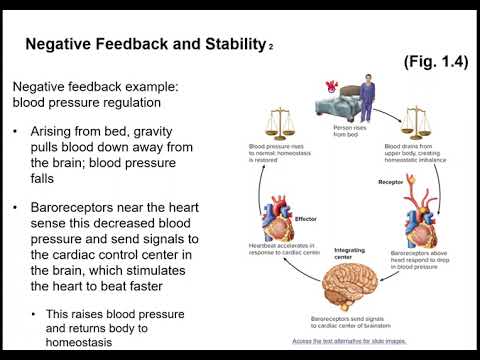The slide, with a white background, presents the concept of negative feedback and stability, specifically focusing on blood pressure regulation as an example. The left side of the slide, under the bold title "Negative Feedback and Stability," details the process in a series of bullet points: 

1. "Arising from bed, gravity pulls blood down away from the brain, causing a drop in blood pressure."
2. "Baroreceptors near the heart sense this decreased blood pressure and send signals to the cardiac control center in the brain."
3. "The cardiac control center stimulates the heart to beat faster, which raises blood pressure and returns the body to homeostasis."

On the right side, labeled as figure 1.4, a clockwise cycle visually represents this process. At the top, an image shows a man standing beside a bed with the caption, "Person rises from bed." An arrow points to the next image of scales, labeled, "Blood drains from the upper body, creating static imbalance." This is followed by an image of a heart, then a brain labeled "Integrating center," indicating where the signals are processed. The cycle continues with another heart image and scales, concluding with "Blood pressure is restored to normal," thus illustrating the negative feedback loop that maintains stability in blood pressure regulation.